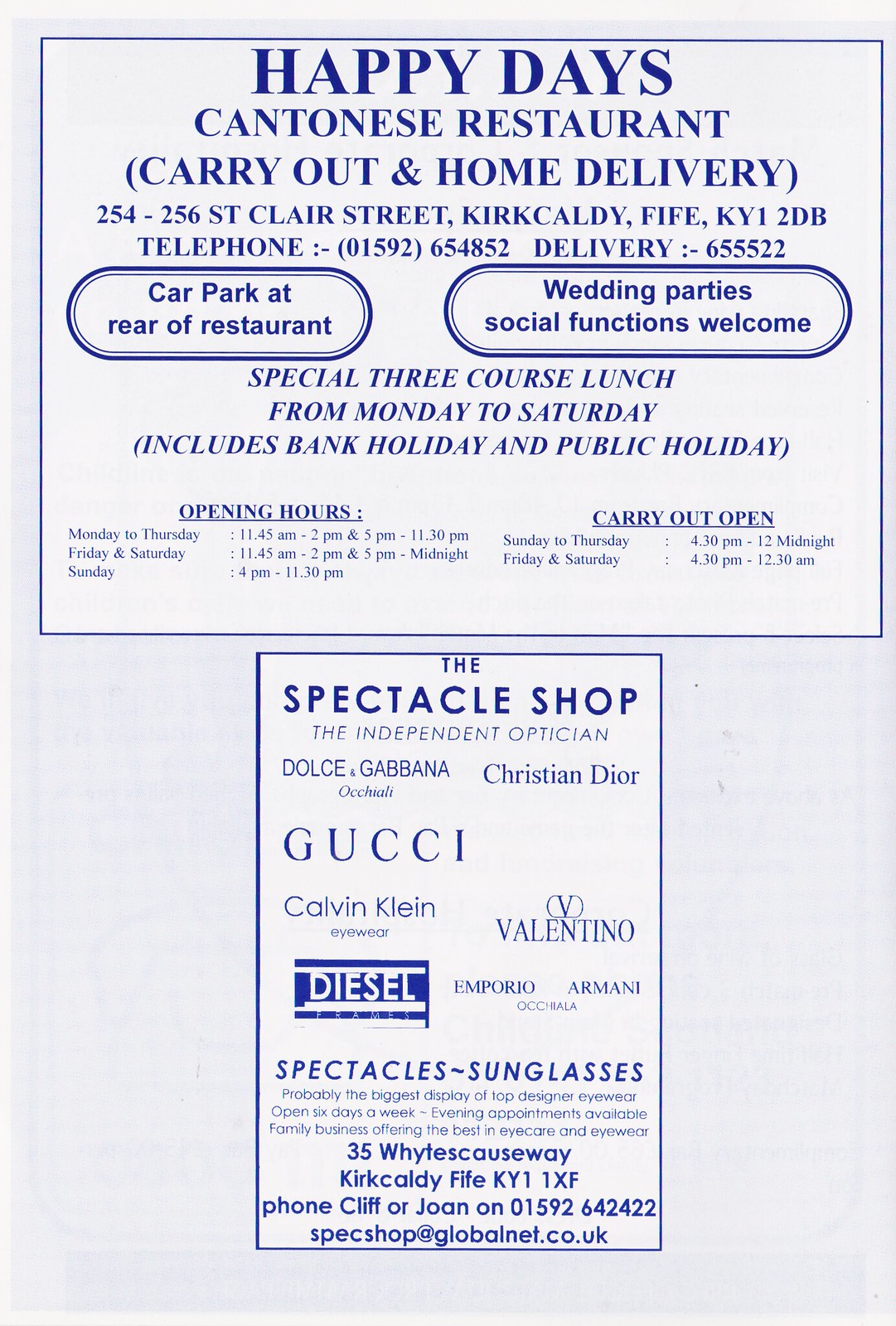This image features what appears to be an advertisement page, possibly from a magazine or a sports program. The page has a gray background with two main ads printed in white and dark blue colors.

At the top of the page, there is a large, horizontally oriented blue rectangle displaying an advertisement for the "Happy Days Cantonese Restaurant." The ad, in blue letters, includes text such as "Carry out and home delivery," the restaurant's address and phone number, and details about available parking at the rear of the establishment. Additionally, the ad mentions that the restaurant accommodates wedding parties and social functions. The ad also lists its operating hours, including a note that they are open on bank and public holidays.

Below this, there is a smaller, vertically oriented blue rectangle advertising "The Spectacle Shop," an independent optician. This ad highlights several designer brands they offer, such as Gucci, Dolce and Gabbana, Christian Dior, Calvin Klein, Diesel, and Valentino. At the bottom of this ad, the store's address, phone number, and email address are provided.